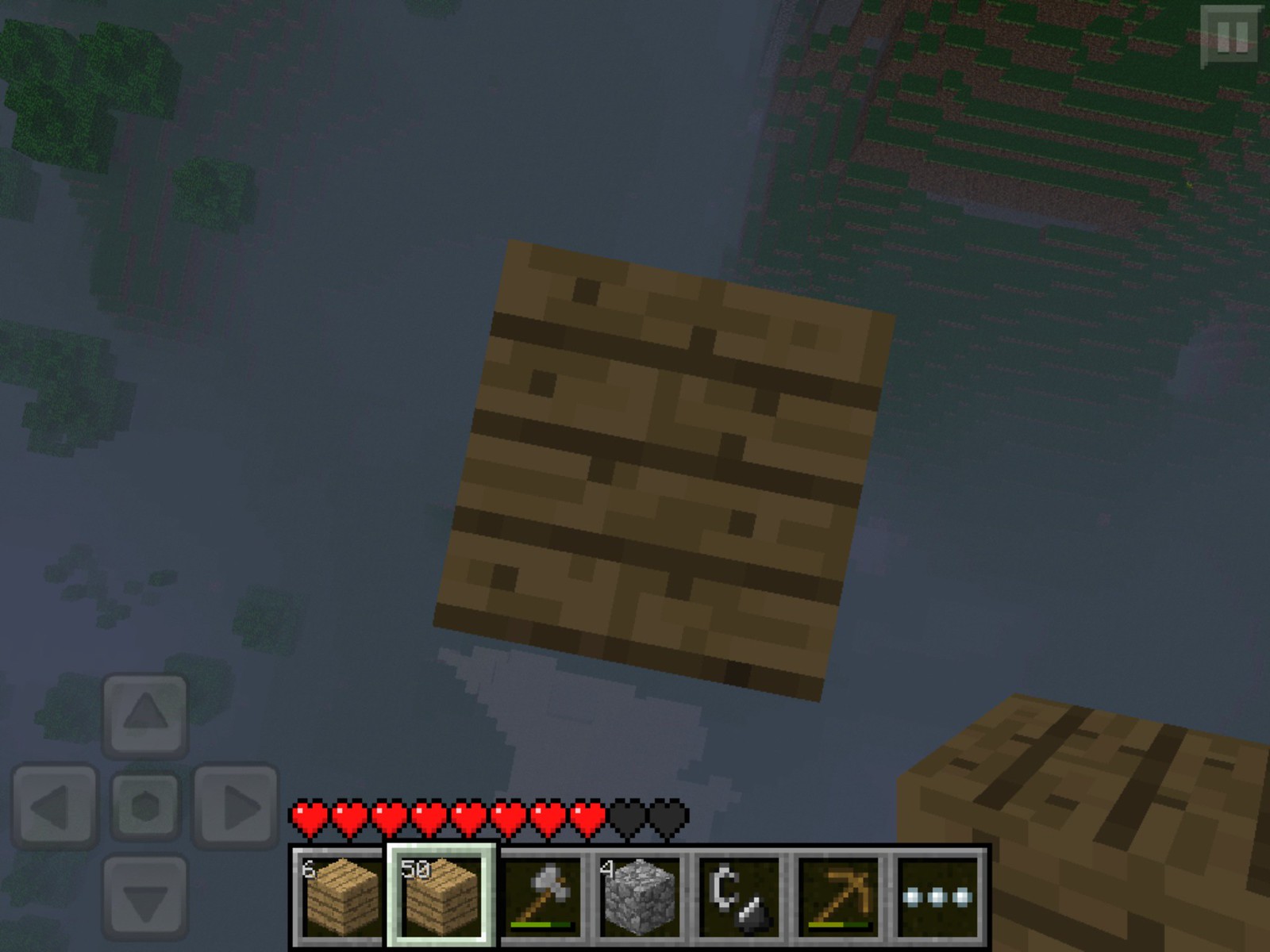This is a screenshot from a mobile version of Minecraft. The image is predominantly dark blue, indicating a water-themed environment. Central to the screen is a slightly tilted wooden block constructed from variously colored squares including shades of brown, light green, and light tan, with dark brown lines dividing it horizontally. Surrounding this block are other similarly styled blocks, some appearing to float or be submerged in water, suggesting reflections or submersion.

The user interface (UI) is evident with a navigational control panel in the lower left corner featuring up, down, left, right arrows, and a central action button with a circle. The game's HUD (heads-up display) at the bottom showcases a row of seven item slots displaying digital images of different items: a crate marked '6', another crate with '50', an axe, a cube, an unknown object labeled '4', a crossbow or pickaxe, and three dots. Above these items, a health indicator shows nine hearts, of which six are illuminated red and two are darkened, implying that the player has lost two lives or hearts. 

In the upper right corner, there are pause controls indicated by two vertical lines, and there may be reflections or additional blocks visible, contributing to the immersive and cubic nature of the game environment. This detailed setup suggests the player’s goal might involve navigating and collecting items from the floating crates while potentially facing various in-game challenges.